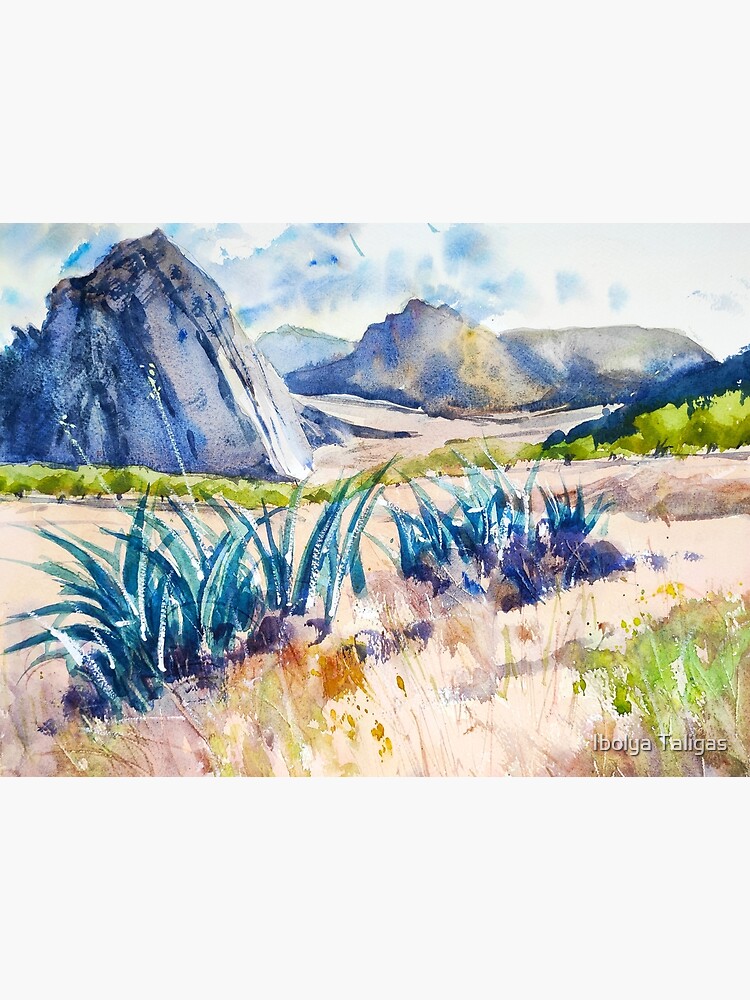This is a detailed watercolor painting of a mountainous landscape with a signature in the bottom right corner, signed by Aibola Talagas or I Bolia Salinas. The background consists of a white sky interspersed with blue and white clouds. Three mountain ranges dominate the composition; the largest and closest mountain sits on the left, characterized by bluish and rocky textures. Below this mountain lies a valley with brown fields transitioning into a horizontal line of small green trees across the painting. 

In the foreground, the viewer is greeted by a variety of plant life: bushes with blue-green hues, tall plants with green leaves, and blossoms resembling dry seed pods. The ground is a mixture of flat grasslands, yellow and brown in color, punctuated with small blotches of paint to mimic grass or additional bushes. Overall, the painting effectively creates a sense of depth, giving the impression of standing at the edge of a valley, gazing towards distant hills and a serene mountainous backdrop.